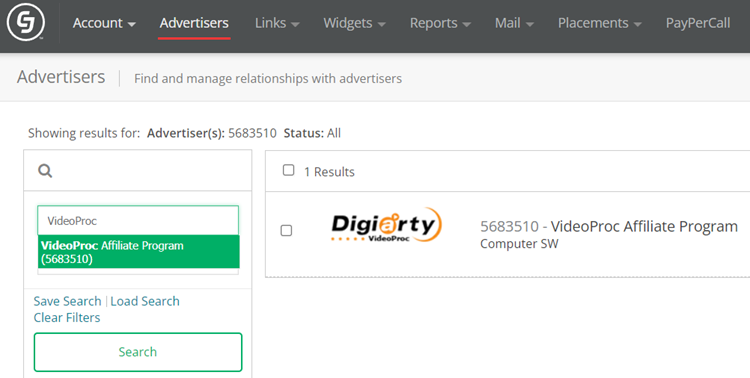This is a detailed screenshot from the AI converter program, Videoproc. The interface features a gray header with several sections, including "Account," "Advertisers," "Links," "Widgets," "Reports," "Mail," "Placements," and "Paper Call." The "Account Advertisers" section is highlighted in white and underlined in red.

Beneath the header is a subtitle: "Advisors find and manage relationships with advertisers." The page displayed is a search results page, listing approximately 56,835,110 advertisers.

There are two main boxes below this text. The left box contains a search section at the top, followed by another box labeled "Videoproc." Within this box is a green-labeled section titled "Videoproc Affiliate Program (5,683,510)." Additionally, it includes hyperlinks for "Save Search," "Load Search," and "Clear Filters," alongside a search button outlined in green.

The right box comprises two checkboxes. The first checkbox, labeled "One result," is selected, whereas the second checkbox remains unchecked. This unchecked box is associated with a product "DigiRT from Videoproc," with the number "5,683,510" next to it. This section also highlights the "Videoproc Affiliate Program Computer SW."